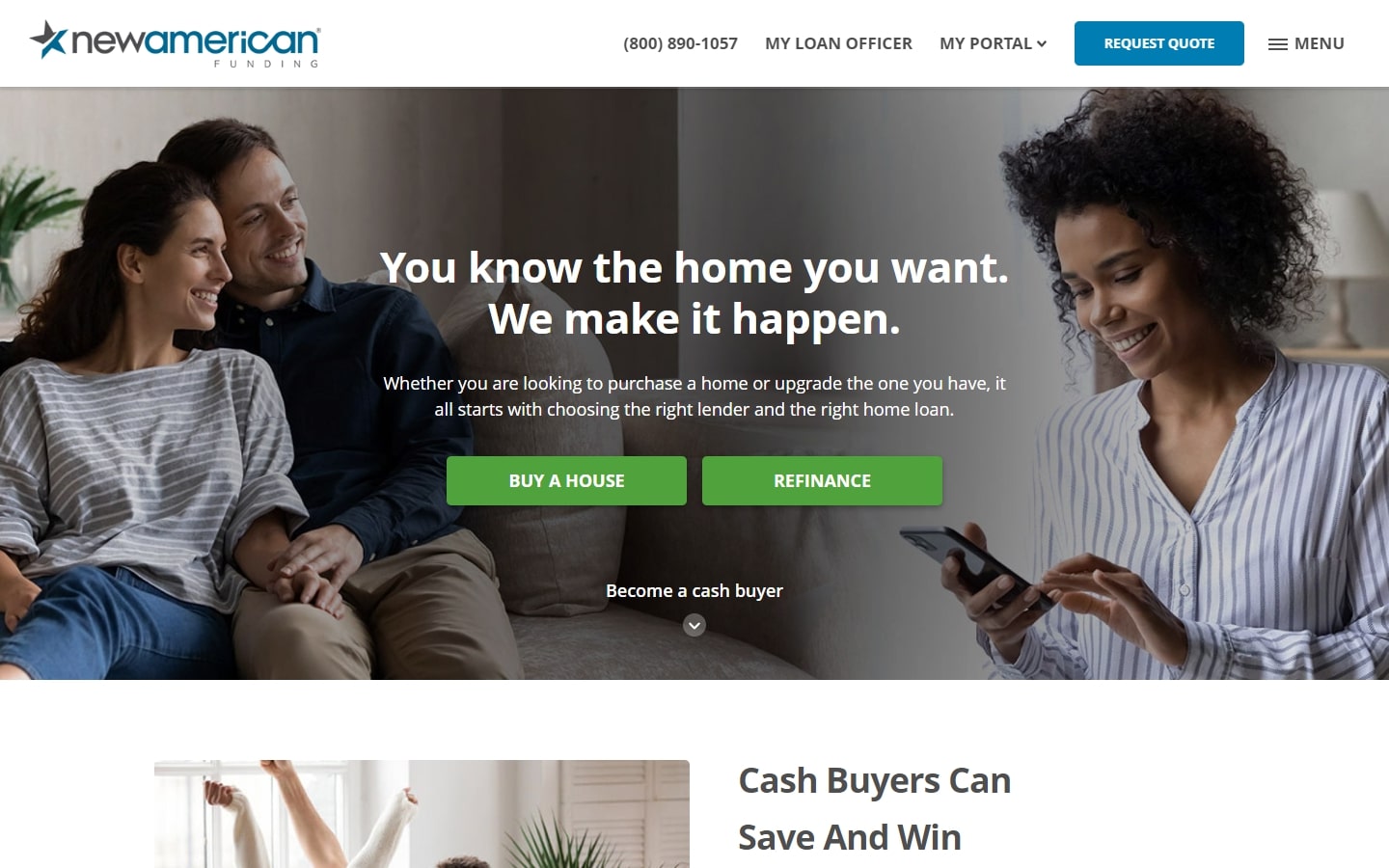The website for New American Funding, a loan service specializing in home purchases and refinancing, features a detailed and user-friendly design. At the top of the page, the company's name is displayed in lowercase, with "new" in dark text and "american" in blue, accompanied by a star logo. To the right, important contact information is provided, including a phone number: (800) 890-1057. Adjacent to this, options such as "My Loan Officer," "My Portal," and "Request Quote" buttons, along with a clickable menu tab, offer easy navigation.

The main image on the homepage portrays a warm and inviting scene: on the left, two people sit close together on a couch, sharing a smile, while on the right, a woman with dark skin, curly hair, and wearing a blue buttoned, long-sleeve shirt, looks down smiling as she dials her cell phone.

Centered within the image, a compelling message reads, "You know the home you want, we make it happen. Whether you are looking to purchase a home or upgrade the one you have, it all starts with choosing the right lender and the right home loan." Below this, two prominent green buttons with white text invite users to "Buy a House" or "Refinance."

Further down, a section titled "Become a Cash Buyer" with a clickable downward-pointing arrow, is visible. Accompanying this section is a small image of hands raised in the air beside a plant. Next to the image, a message reads, "Cash Buyers Can Save and Win," highlighting the potential benefits of becoming a cash buyer.